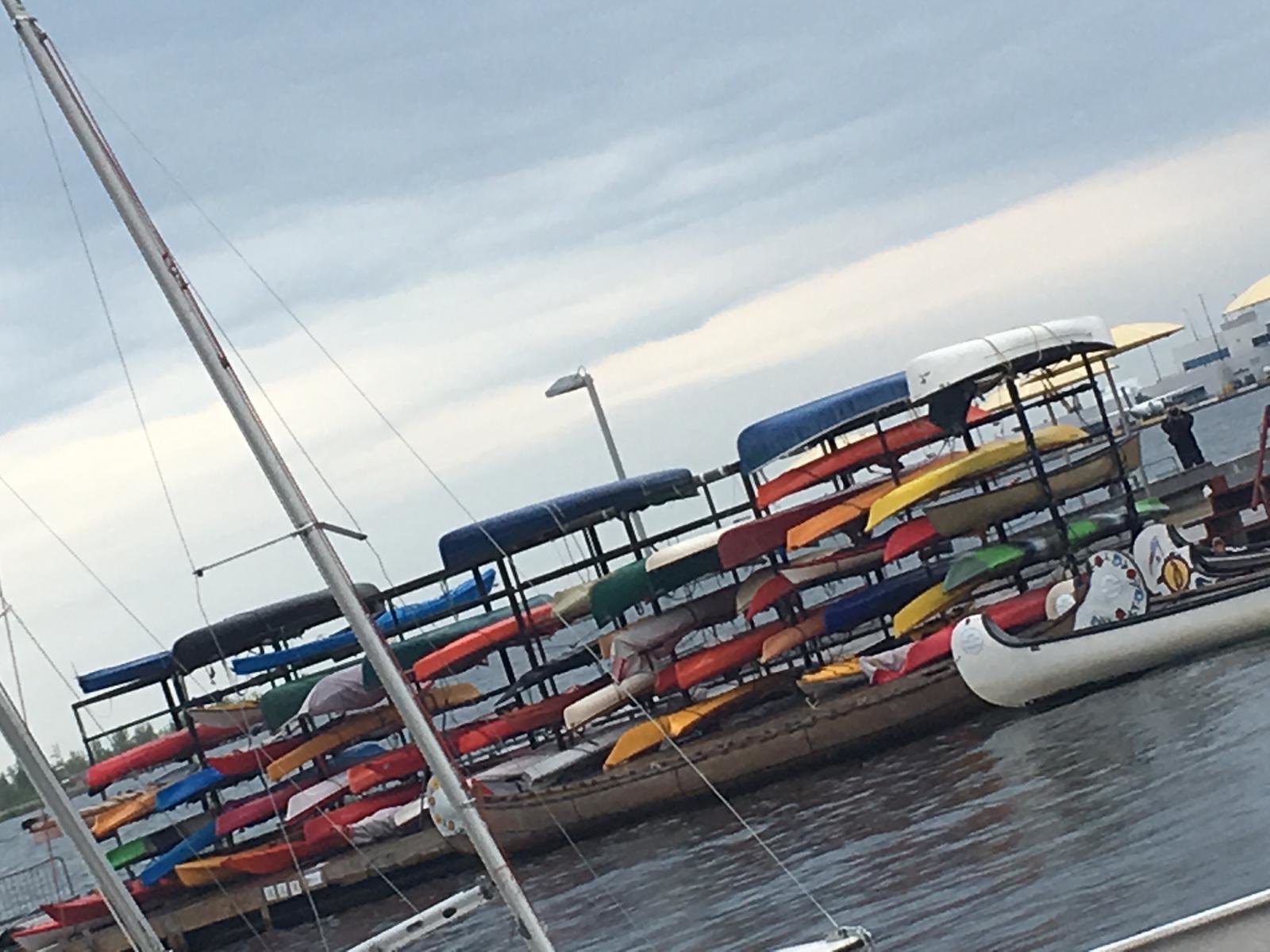This photograph captures a tilted daytime scene taken from a boat, showcasing a calm lake surface with faint, choppy waves against a backdrop of hazy, cloudy skies. The upper half of the image is dominated by a gray sky with patches of brighter clouds. In the left edge of the background, there are some trees that outline the shoreline. The central subject is a long, brown boat equipped with metal racks holding an array of colorful kayaks and canoes—red, yellow, white, blue, black, and orange—all stored upside down in rows, with seven layers of boats stacked from top to bottom. A streetlight-style lamp is mounted on the boat, presumably for nighttime illumination. In the distance, a figure, possibly a man, stands on what appears to be a dock in the middle of the water. The entire scene is set against a serene and hazy atmosphere, hinting at a secluded lakeside location.